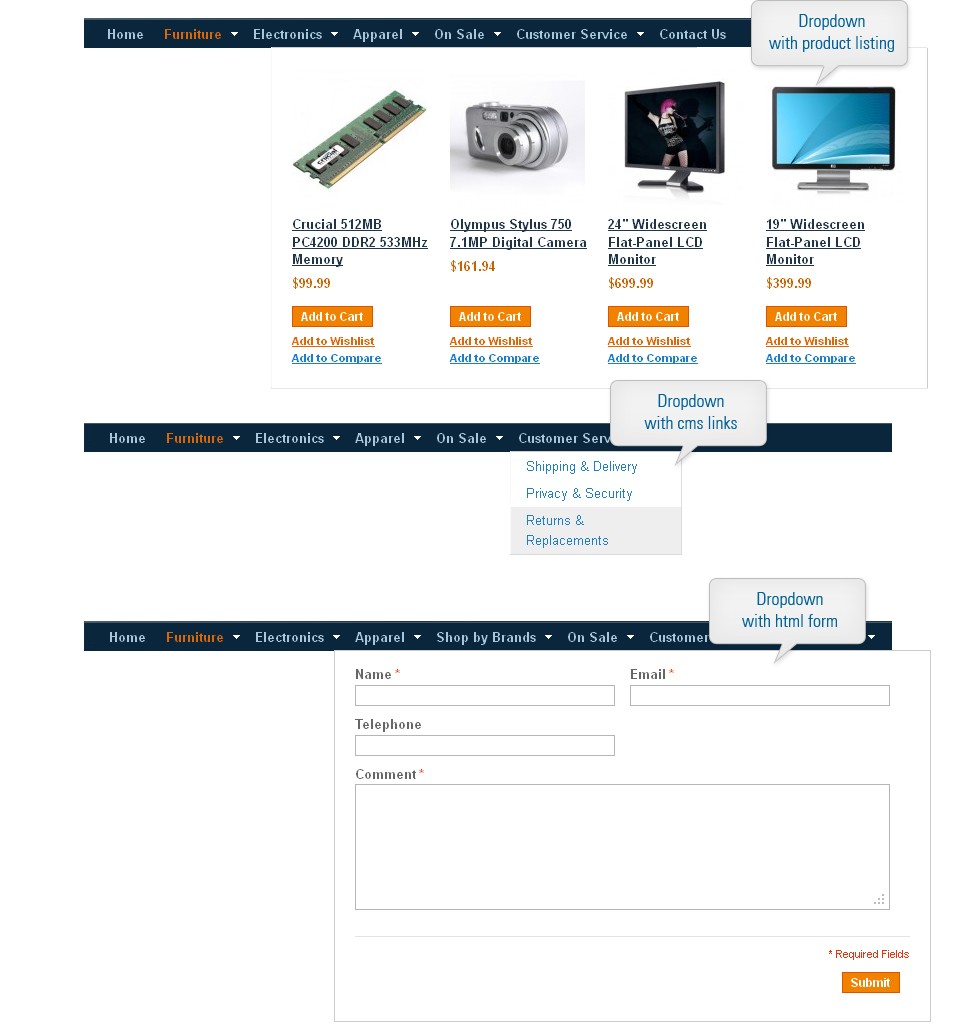The image showcases a comprehensive web page layout specifically designed for an online store. At the very top left corner of the page, there is a navigation menu starting with "Home". Adjacent to "Home" is "Furniture" displayed in striking orange text, followed by "Electronics", "Apparel", "On Sale", "Customer Service", and "Contact Us".

On the top right corner, there's a gray background rectangle labeled "Drop Down with Product Listing". 

Beneath this section, the page displays images of various products in a horizontal arrangement. The first image features an electronic component, followed by a digital camera to the right. Next in line is a flat screen monitor, and lastly, a flat panel monitor. Below each product image, the price is prominently displayed, accompanied by an orange "Add to Cart" button, as well as options to "Add to Wish List" and "Add to Compare".

Further down, there is a black rectangular section containing a repeated sequence of navigation links: "Home", "Furniture" highlighted in yellow, "Electronics", "Apparel", "On Sale", and "Customer Service". Under "Customer Service", sub-categories such as "Shipping and Delivery", "Privacy and Security", and "Returns and Replacements" are listed.

A secondary navigation bar below these categories adds an extra link, "Shop by Brands", to the initial menu set: "Home", "Furniture", "Electronics", "Apparel", "On Sale".

Towards the bottom of the page is a form layout featuring several text boxes for user input: "Name", "Email", "Telephone", and a larger box labeled "Comment". At the very bottom is a prominent "Submit" button, inviting users to send their information.